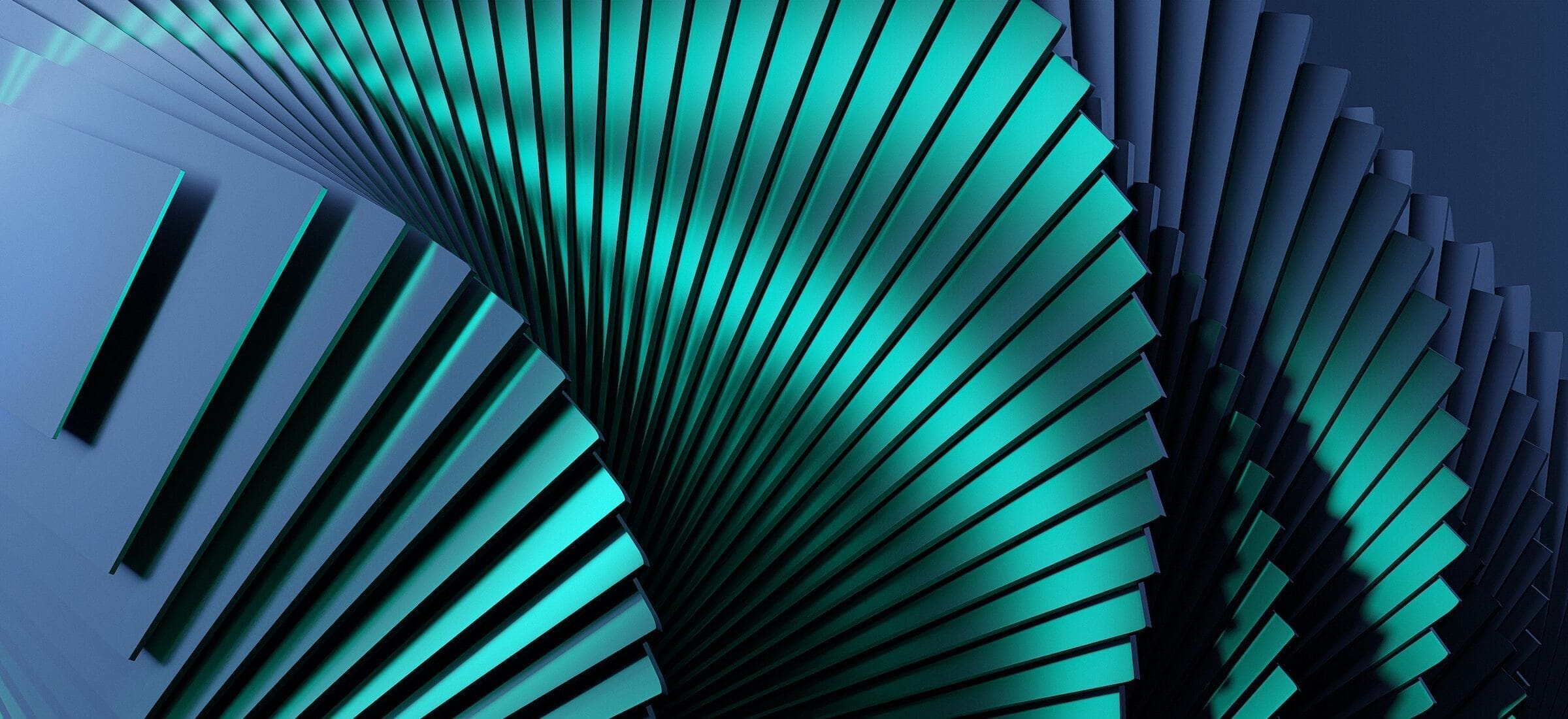This detailed illustration or digital rendering presents a highly abstract and visually striking 3D composition, resembling a series of spiraling stairs or stacked metallic sheets. The design features five rows of winding, accordion-like steps that transition fluidly from a dark navy blue at the top to a teal aquamarine hue as they fan out. The central staircase appears the longest, encompassing approximately 40 steps. These reflective stairs alternate between darker and lighter shades of blue, creating a dynamic visual effect as light interacts with the metallic, shiny surface. The entire formation stands out against a matching dark blue background, enhancing the contrast and depth of the piece. The intricate blend of colors and textures gives the impression of a sophisticated, layered sculpture, evocative of fanned-out post-it notes or accordion patterns, skillfully capturing both movement and stillness in its design.